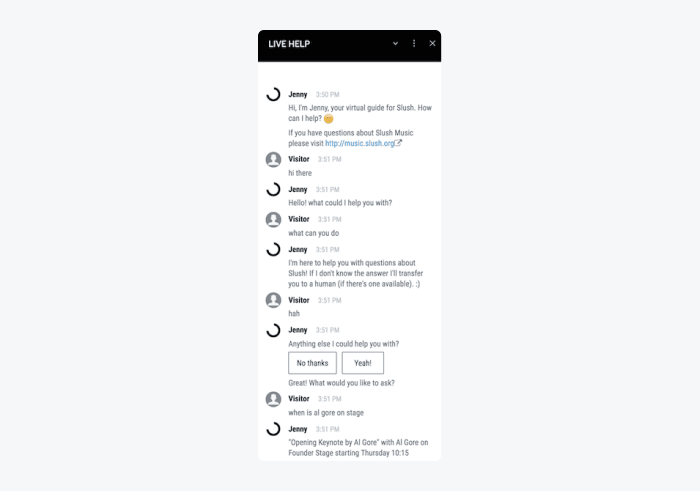The image portrays a live chat window with a black background, titled "Live Help" at the top. On the top-right corner, there are three icons: a down arrow, three vertical dots, and an 'X' button for closing the chat. The conversation displayed in the chat is as follows:

- **Jenny (3:50 PM):** "Hi, I'm Jenny, your virtual guide for Slush. How can I help you? 🙂 If you have questions about Slush Music, please visit [http://music-clutch.org](http://music-clutch.org)."
- **Visitor (3:51 PM):** "Hi there"
- **Jenny (3:51 PM):** "Hello, what can I help you with?"
- **Visitor (3:51 PM):** "What can you do?"
- **Jenny (3:51 PM):** "I'm here to help you with questions about Slush. If I don't know the answer, I'll transfer you to a human if there's one available."
- **Visitor (3:51 PM):** "Huh?"
- **Jenny (3:51 PM):** "Anything else I could help you with?"
- The options presented are "No thanks" or "Great, what would you like to ask?"
- **Visitor (3:51 PM):** "When is Al Gore on stage?"
- **Jenny (3:51 PM):** "Opening keynote by Al Gore on Foundry's stage starting Thursday at 10:15 PM."

The conversation shows Jenny, a virtual guide, assisting the visitor with questions related to the Slush event, mentioning an upcoming keynote by Al Gore.